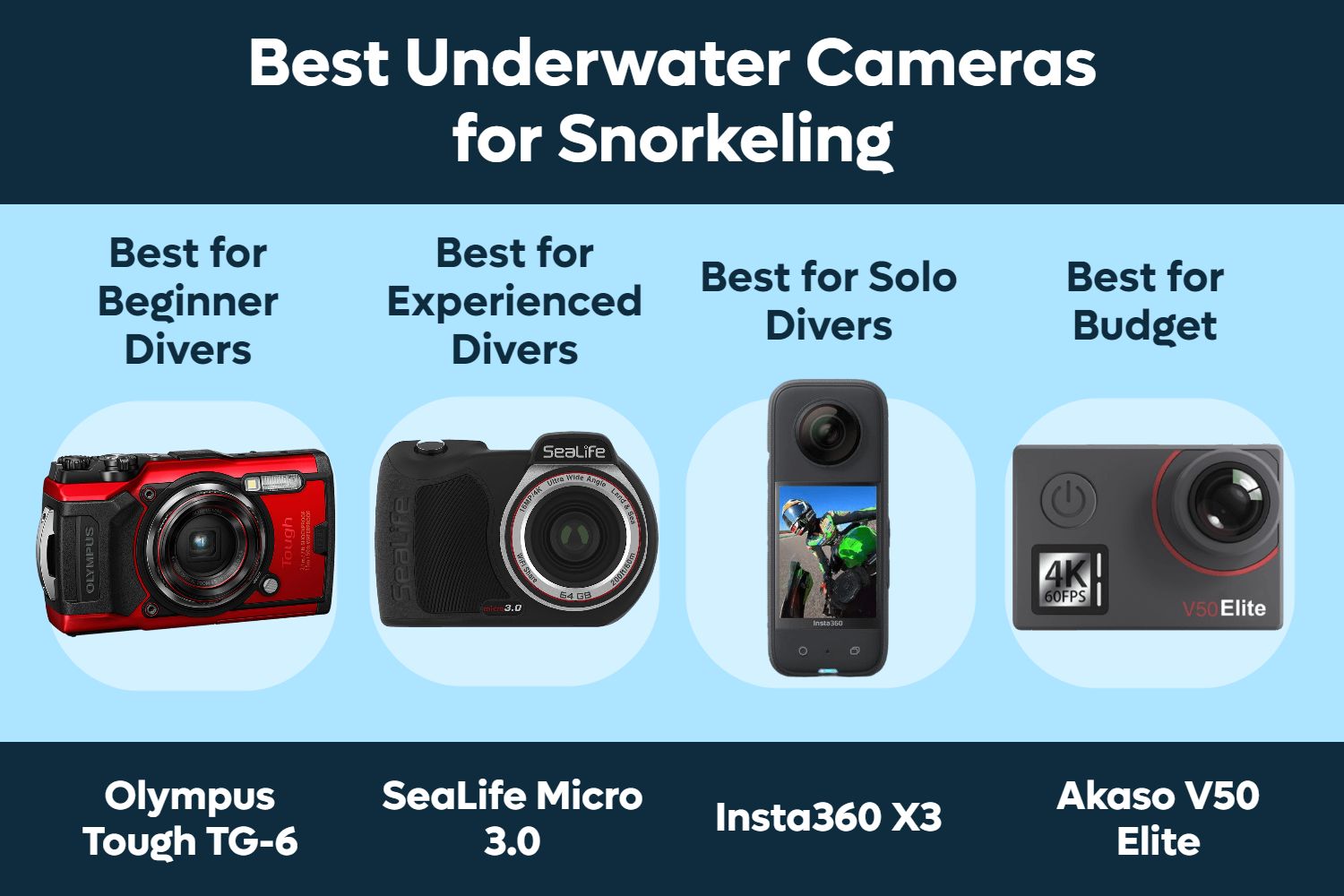The image is a detailed advertisement poster showcasing the best underwater cameras for snorkeling. At the top of the poster, within a dark blue text box with bold white letters, it reads "Best Underwater Cameras for Snorkeling." Below, on a baby blue background, four camera models are highlighted:

1. **Olympus Tough TG-6**: A red and black camera labeled “Best for Beginner Divers,” featuring an industrial and beefy design.
2. **SeaLife Micro 3.0**: A black camera with a metallic center around the lens, noted as “Best for Experienced Divers.”
3. **Insta360 X3**: A thin, rectangular-shaped black camera resembling a smartphone, identified as “Best for Solo Divers.”
4. **Akaso V50 Elite**: A rectangular camera with a matte gray finish and a prominent power button, described as “Best for Budget.” 

Each camera model has its name and designation displayed in dark blue text boxes with white text underneath the respective camera images.